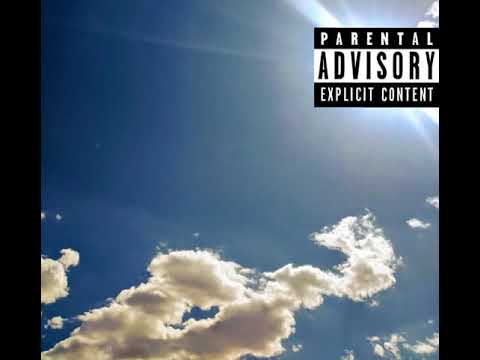The image depicts the cover of a CD, prominently featuring a "Parental Advisory Explicit Content" label in the upper right corner. The label consists of three sections: the top has white text on a black background reading "PARENTAL," the middle has black text on a white background reading "ADVISORY," and the bottom has white text on a black background reading "EXPLICIT CONTENT." Flanking the cover, there are vertical black lines running top to bottom on both edges. The main image showcases a vivid sky transitioning from a dark blue in the upper left to a lighter blue as it moves toward the sun in the upper right. Situated behind the parental advisory label, the sun shines brightly, with rays of light emanating, particularly towards the upper left and lower right. Beneath the sky, puffy clouds start from the lower left, gradually transitioning from grayish tones in the middle to whiter hues as they spread upwards and to the right. The overall scene, framed by the contrasting black lines, creates a dynamic and visually striking CD cover.